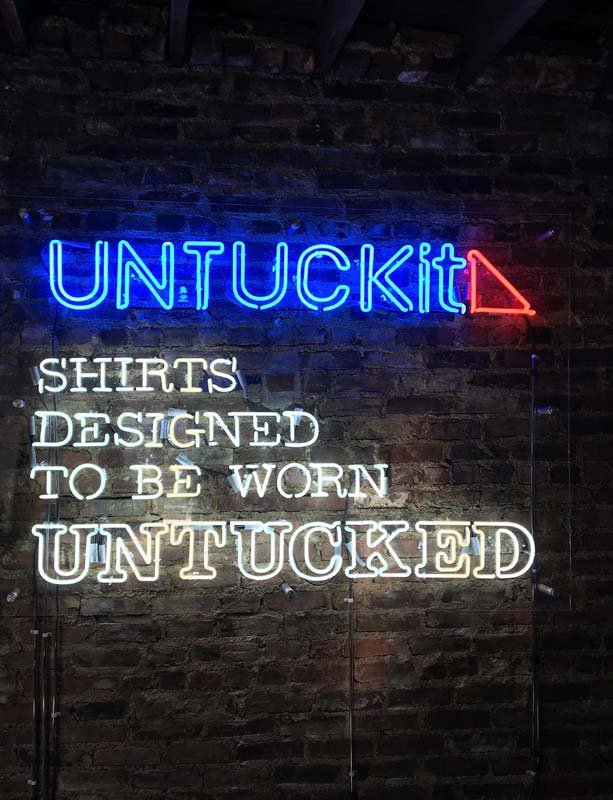This photograph captures a vividly glowing neon sign affixed to a brick wall, advertising the company "Untuck It". The name "UNTUCK IT" is rendered in bright blue bubble neon lights, immediately followed by a sharp red neon triangle. Positioned just below this, the company's motto "SHIRTS DESIGNED TO BE WORN UNTUCKED" is displayed in white neon lettering, with "UNTUCKED" also in the same distinctive blue bubble style as the name above. The image appears to be taken in a dimly lit space, possibly suggesting the ambiance of a comedy club or similar venue, but the neon sign itself radiates brightly against the rustic brick backdrop, highlighting the worn yet striking aesthetic of the advertisement.